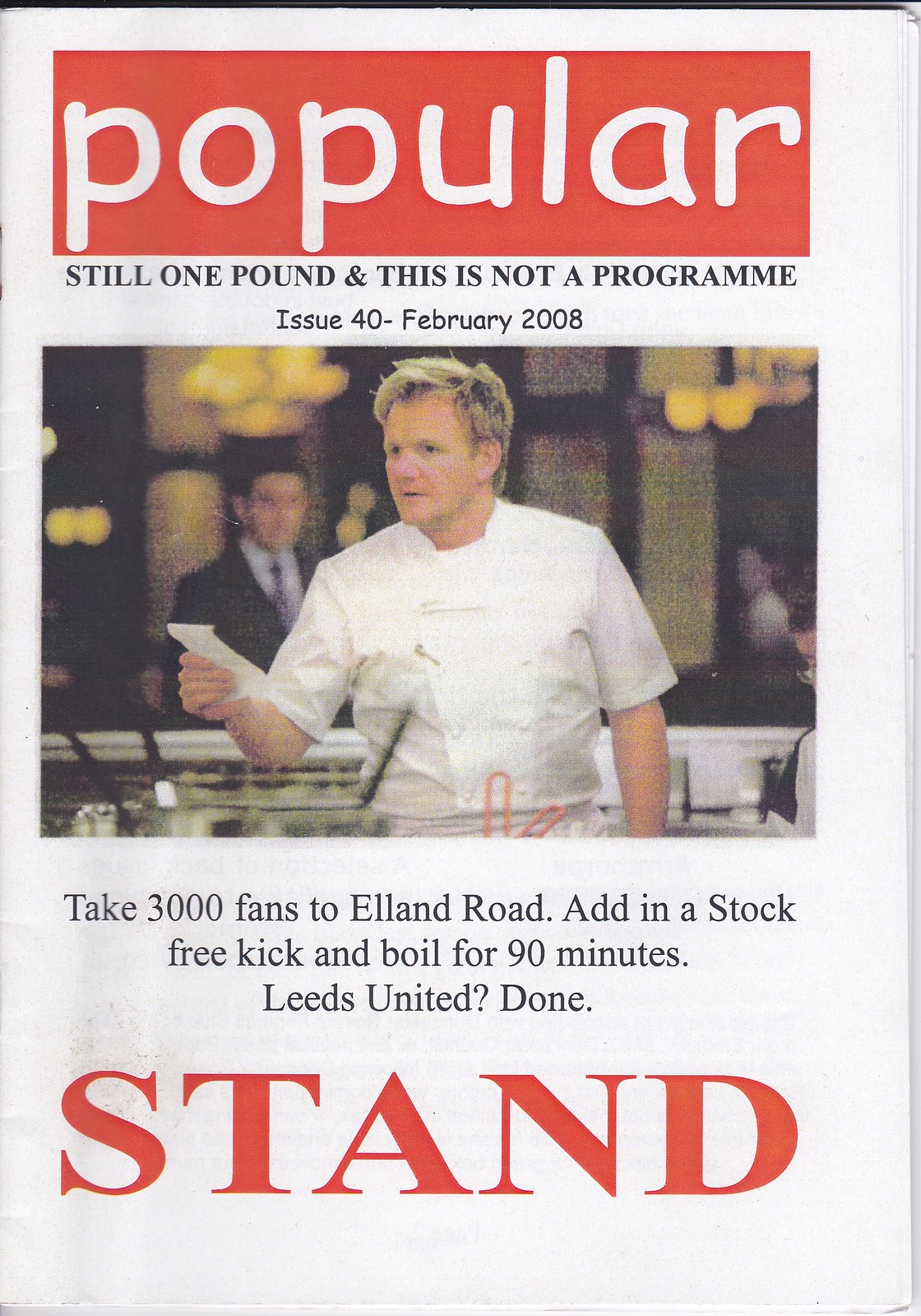The image is a vertical rectangular magazine cover predominantly featuring a large red band at the top with the word "Popular" in white Comic Sans-style text. Below this red band, the cover has text in black stating, "Still One Pound" and "This Is Not a Program," along with "Issue 40 - February 2008" in smaller letters. At the center of the cover, there is a photograph of Gordon Ramsay, assumed to be taken from the show "Hell's Kitchen." In the photo, Ramsay is in what appears to be a kitchen within a restaurant setting; a man stands over his shoulder looking at the camera, and there are visible restaurant patrons in the background seated at a table. The colors featured on the cover include white, black, red, yellow, grey, and orange. At the bottom, there is a humorous segment related to football, encouraging fans to "take 3,000 fans to Elland Road, add in a stock-free kick, and boil for 90 minutes, Leeds United, done" followed by the word "Stand" in large red text.